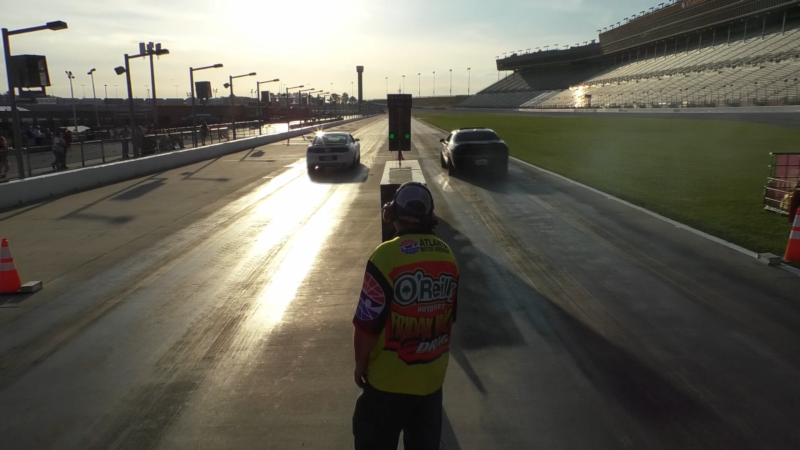This detailed color photograph captures a vibrant scene on an outdoor drag racing track under a blue sky with a sun-bleached patch. In the foreground, a man stands with his back to the camera, dressed in a distinctive yellow t-shirt featuring black and red trim, and adorned with advertisements, including "Atlanta," "O'Reilly," and a partially readable "Friday Drag." He's also wearing a cap and headphones. Directly in front of him is a machine displaying stop-and-go lights, with the green light currently illuminated, indicating the starting point for the race.

On the track, two cars are positioned and ready to race - a white car on the left side and a black car on the right side. Both vehicles are seen from the rear. On the far left, there is a visible cone, a strip of cement curb, followed by a white wall, and a series of street lamps. There are also onlookers gathered on this side of the track. To the right of the roadway lies a grassy area, beyond which are the empty spectator stands of the stadium. This setup presents the anticipation of a drag race about to commence.